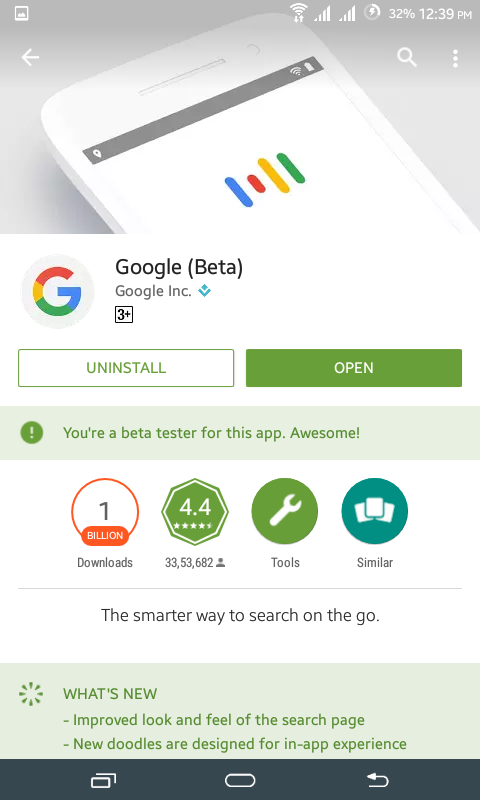This screenshot captures a Google beta test screen with a variety of detailed features. In the middle of the screen, there is a prominent green information bar indicating that the user is a beta tester for this app. The screen presents options to either open the app or uninstall it.

Highlighted in the upper section is a red circle containing the number "1" followed by the word "billion," signifying that the app has reached one billion downloads. Additionally, the app boasts a commendable rating of 4.4 stars based on reviews from 3,353,682 users.

To the side, there is a green tool button icon, presumably for accessing further options or settings. Nearby, a circular section displays three similar apps, providing users with quick access to alternatives.

A descriptive text below the similar apps section reads: "The smarter way to search on the go," emphasizing the app's efficiency and convenience.

Towards the bottom of the screen, within a green box titled "What's New," updates are itemized, mentioning improvements to the look and feel of the search page and the introduction of new doodles designed for an enhanced in-app experience.

At the top of the page, there's an image of a smartphone displaying the iconic Google search listening bar with its recognizable blue, red, yellow, and green colors. The phone's information bar is visible at the topmost part of the screen, showing signal strength, open applications, and other standard phone indicators.